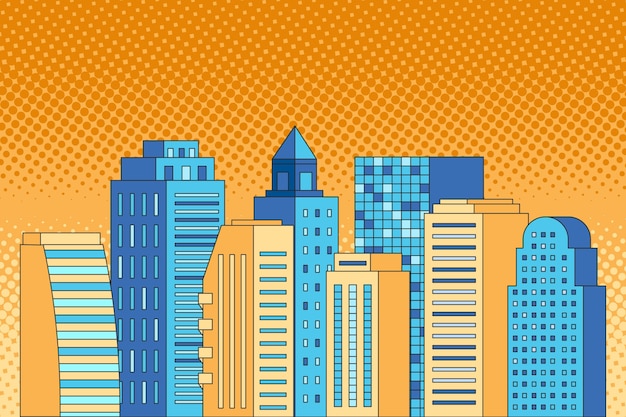This image is a digital, cartoonish depiction of a vibrant city skyline, characterized by an array of eight skyscrapers in various shapes and colors. The buildings, each adorned with numerous windows in square, lengthwise, and dot patterns, alternate between shades of blue and orange, with some displaying golden hues. The contrasting colors create a striking pattern. The background transitions from orange at the top to yellow towards the bottom, sprinkled with small, dark gold dots throughout, adding depth and texture to the scene. The artistic rendering captures the whimsy and dynamism of an urban landscape through its playful use of colors and shapes.